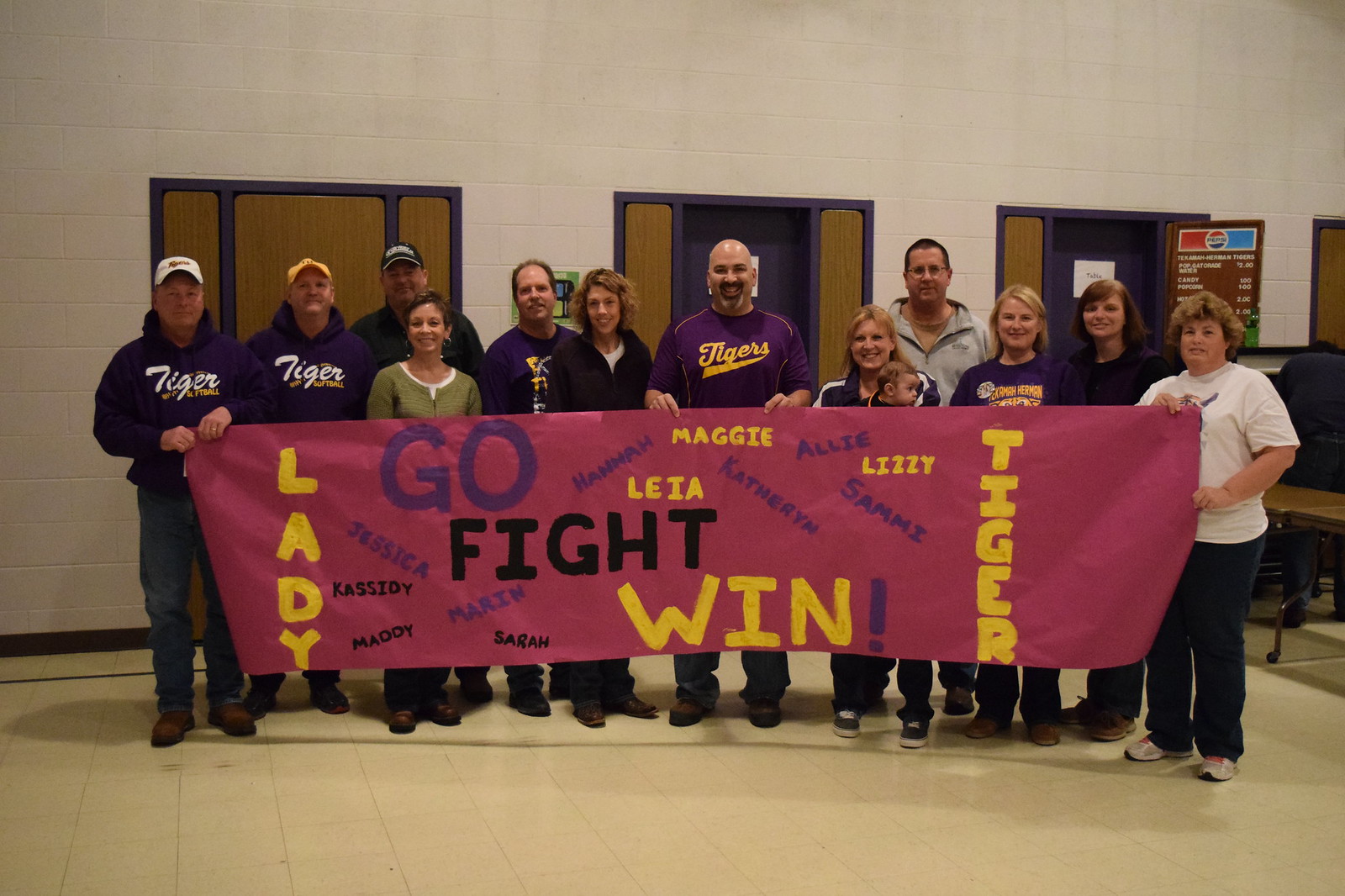In this horizontally oriented photograph taken inside a large room with a white brick-shaped wall, a group of approximately 13-15 adults is showcased. They stand on a beige-tiled floor in front of three brown doors, with the left door closed and the middle and right doors open. Notably, the door on the right displays a Pepsi logo sign with prices visible, suggesting a cafeteria setting. 

The group is holding a long, paper banner with a dark red or purple background. Vertically written on either end of the banner are the words "Lady" and "Tiger" in yellow letters. The center of the banner prominently displays the words "Go," "Fight," and "Win" in purple, black, and yellow all-caps letters respectively. Scattered around these central motifs are various names such as "Maggie," "Leah," "Allie," and "Lizzie," seemingly belonging to team members.

The adults holding the banner, likely part of a girls' team, are clad in matching dark purple hoodies with the word "Tiger" written in white on the center. A standout figure among them is a bald man with facial hair, positioned centrally and wearing a jersey-like top that says "Tigers" in yellow. The image seems to capture a celebratory or team spirit moment, possibly within a gymnasium setting conducive to school sports activities.